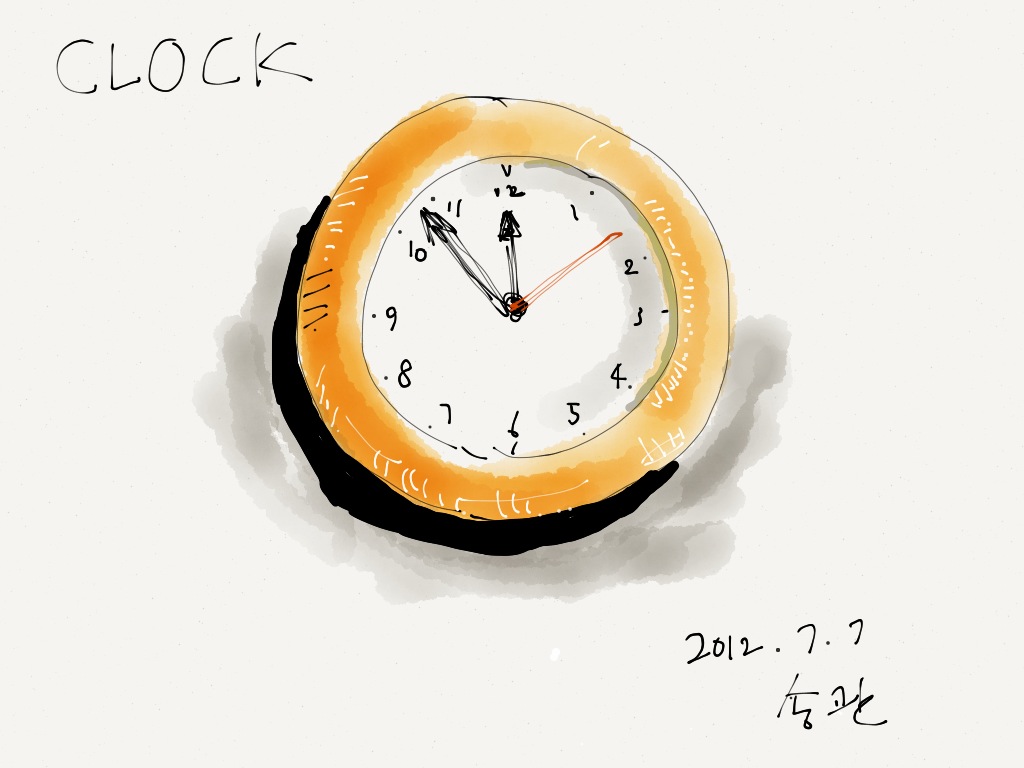This is a detailed hand-drawn illustration, seemingly created with a magic marker, depicting a wall clock. The clock hangs on a stark white wall and prominently features a circular face with a vibrant orange hue, although it may appear gold in different lighting. The clock’s base is black, contrasting sharply against the bright face. The hour, minute, and second hands are marked in black, with the second hand distinctively colored in red. The clock shows the time as 11:51, indicating 9 minutes until noon or midnight. Black text accompanies the illustration, stating "CLOCK." Below this, there is a date stamp: "2012.7.7," and an indistinct signature, hinting at the artist's identity. The entire caption is written in English, providing a linguistic context for the viewer.